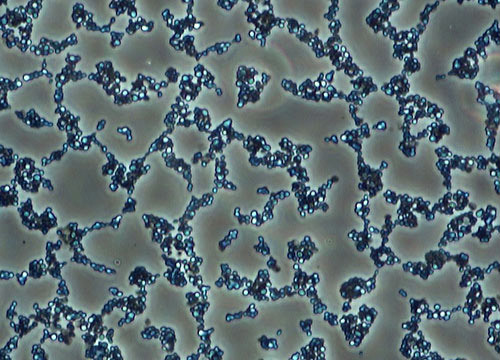This image captures a magnified view through a microscope, likely of germs, bacteria, or organic material clustered together on a slide. The scene is filled with tiny round shapes in various shades of blue, from dark to light, and some white dots. These shapes form irregular clusters and strands that glow slightly, as if illuminated. The background is a bluish-gray color, and each object appears to have a light halo around it, enhancing the impression of microscopic observation. Some areas show single dots scattered throughout, while others display tightly packed bundles and branching patterns, adding to the complexity of the image. In the bottom left-hand corner, a few specks of what appear to be dust can be seen, further hinting at the microscopic nature of the scene.